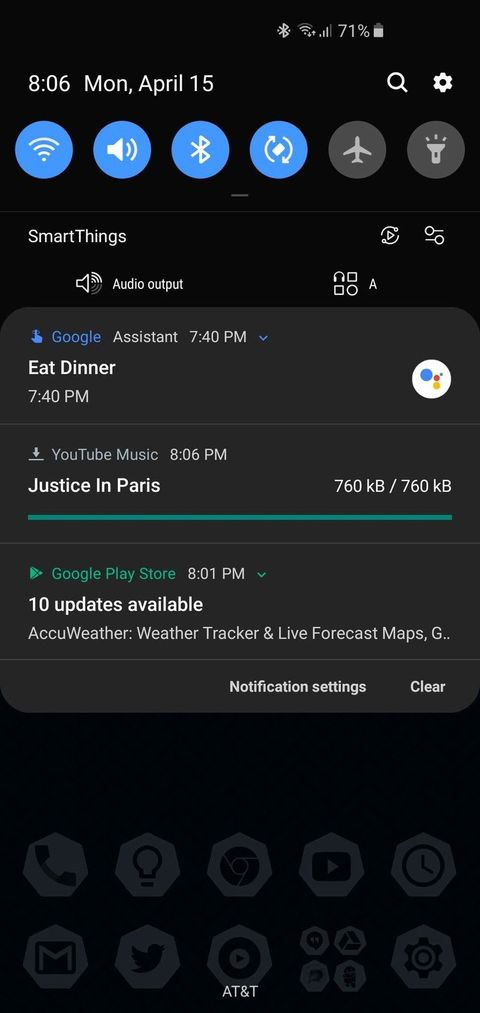Here is a cleaned-up and detailed caption for the image:

On a black background, the screen displays various information and icons. The screen brightness is set to 71%, and the current time is 8:06 PM on Monday, April 15. At the top, there is a magnifying glass and settings icon. Below these are six icons, with the first four being blue and the remaining two gray. These icons include a Wi-Fi signal, a microphone, a Bluetooth signal, and another icon that appears to be a rectangle turned diagonally with arrows forming a circle — likely indicating data sync. Additionally, there are icons for airplane mode and a flashlight. 

Under these, there is a section labeled "Smart Things" featuring a speakerphone, audio output, and Google Assistant (with "Google" in blue while the rest are in white). At 7:40 PM, there is a reminder to eat dinner, followed by "YouTube Music" at 7:40 PM, and "Justice in Paris" at 8:06 PM. The screen also shows that a file of 760 KB has been downloaded completely. 

The Google Play Store icon is displayed in green, indicating that at 8:01 PM, there are 10 updates available. Specific notifications include "AccuWeather: Weather Tracker and Forecast Maps". At the bottom of the screen, there are icons representing various apps, with the first being a phone and the second a light bulb, among a total of ten logos.